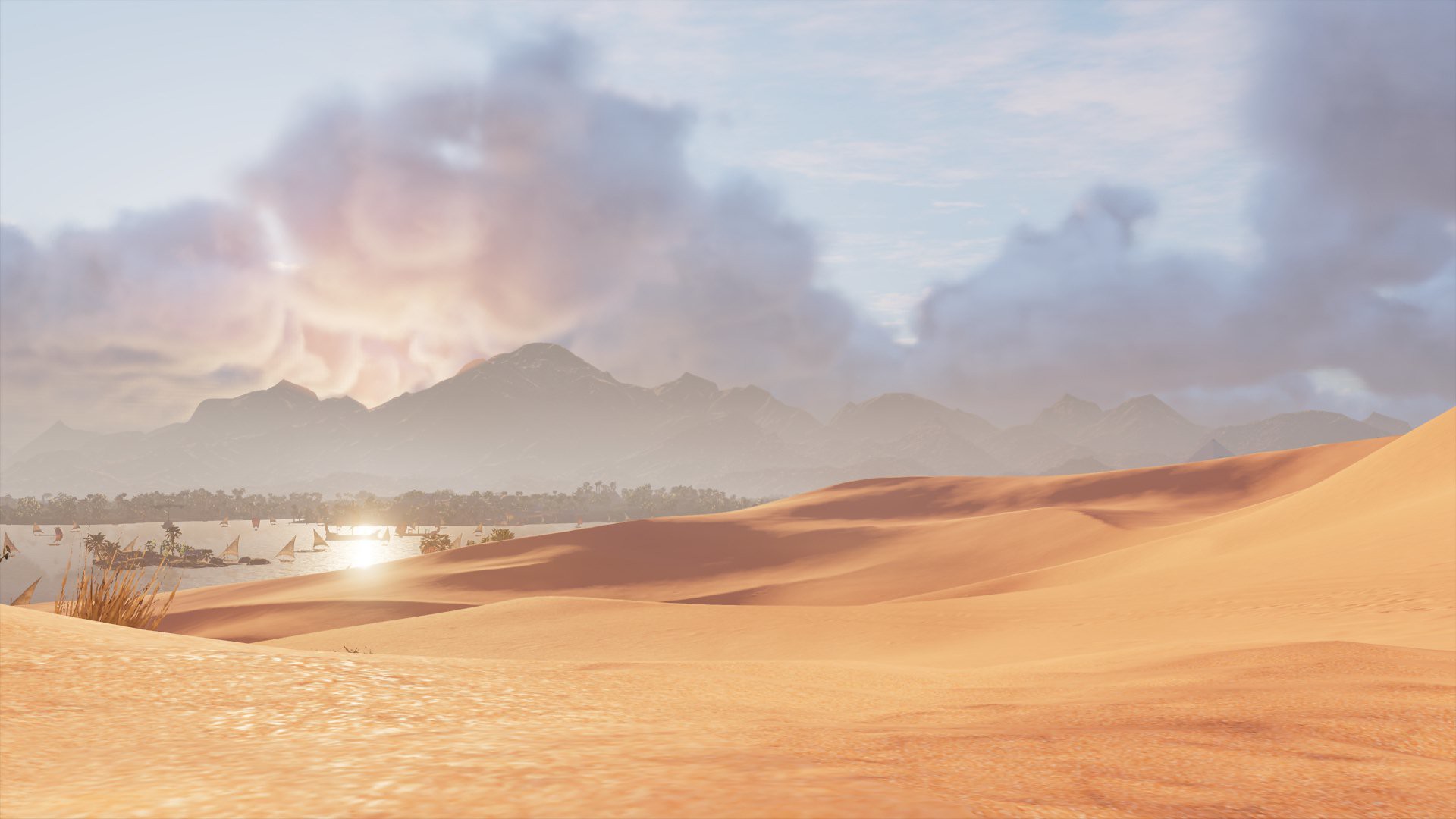This artwork portrays a breathtakingly beautiful sandy beach, so striking it seems almost surreal. The scene features a dreamy coastline on the left, dotted with small sailboats and an idyllic area designed for tourists. A small island is also visible in this section. In the distance, a lush tree line accentuates the tranquil ambiance, evoking images reminiscent of exotic locales such as Polynesia or Malaysia. The sand dunes, with their stunning reddish-brown hues, appear almost too perfect, hinting at artistic enhancement if this were a photograph.

The background presents an ethereal mist shrouding what appear to be volcanoes, creating a foggy, mystical atmosphere. The sun casts its glow flawlessly across the water, adding a warm, enchanting light to the serene setting. Puffy clouds, resembling cotton balls, fill the sky, obscuring the sun's direct rays yet allowing its reflection to dance upon the water, particularly on the left side beyond the sundrenched sands and in front of the imposing mountains.

Whether this is a beautifully executed painting or a dramatically edited photograph, the result is an exquisite, dreamy scene that captivates the essence of a paradisiacal beach surrounded by natural splendor and tranquility.